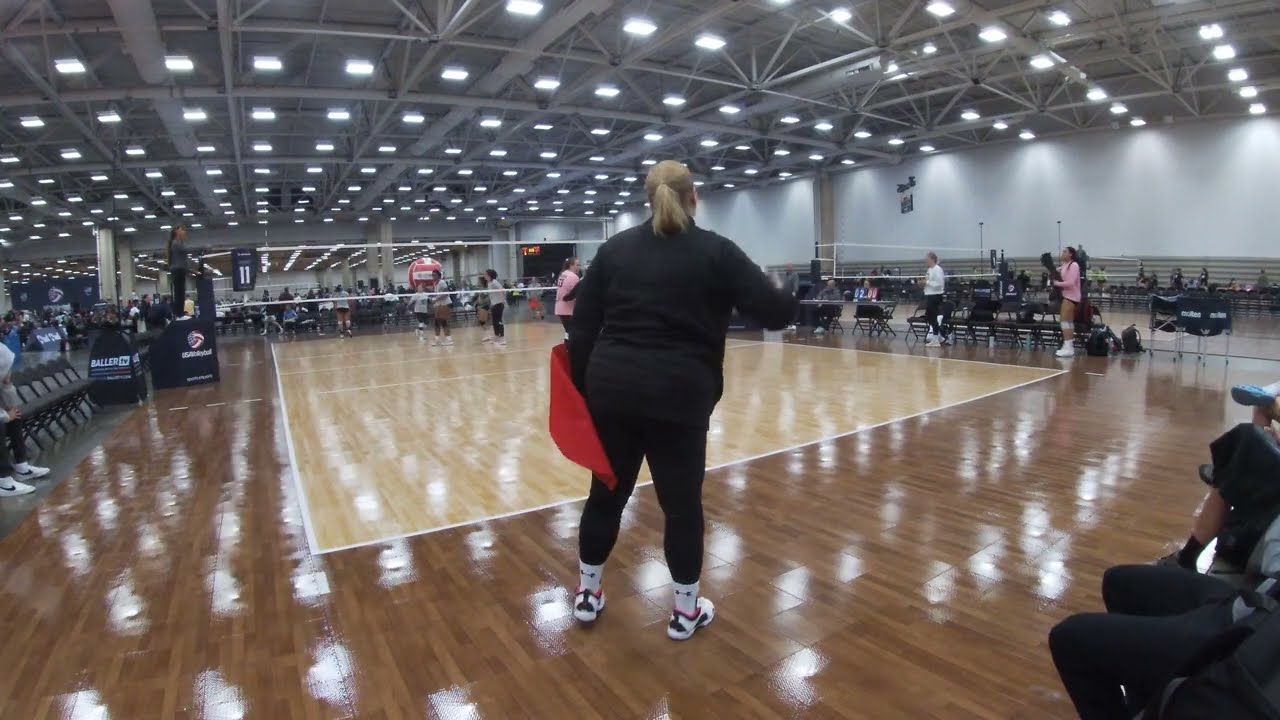The image depicts a bustling indoor gymnasium with a high ceiling adorned with light gray scaffolding and a multitude of rectangular white fluorescent lights that cast a bright, reflective glow on the shiny wooden floor below. This highly polished floor features a volleyball court marked by a light tan rectangle edged with dark brown wood.

At the center of the volleyball court stands a woman of Caucasian descent, wearing a long-sleeved black shirt, black pants, white socks, and black-and-white tennis shoes. Her blonde hair is pulled back into a ponytail. She appears to be preparing to serve, with a volleyball—a mix of red and white—held in her right hand, which is in motion, indicating she might be about to toss it for the serve. In her left hand, she holds a red flag.

Around the court, there are people sitting in chairs on both sides, attentively watching the game. Visible in the far background, a team dressed in white tops and black shorts is mingling, suggesting the match is either about to start or already underway. The entire scene is illuminated by the lights reflecting off the floor, creating a vibrant and active atmosphere typical of a well-lit, indoor sports event.